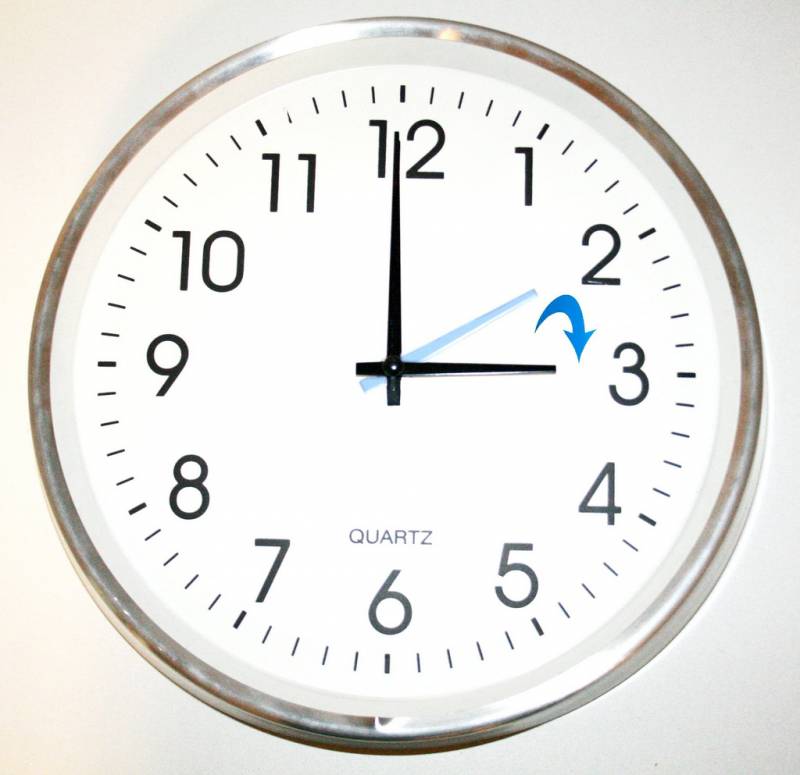This image features a classic wall clock with a sleek silver border surrounding a white face. Prominently displayed are large, black numbers, clearly indicating the time set at 3:00. The clock also includes a light blue diagram of an additional hand, accompanied by a curved arrow pointing downwards toward the right, illustrating the motion of the clock hands. Situated above the number six, the word "Quartz" is noted, signifying the clock's mechanism. Additionally, there's a noticeable small dent directly below the six on the silver frame. At the top-center of the clock, light reflects off the silver border, adding a touch of brightness from the background.